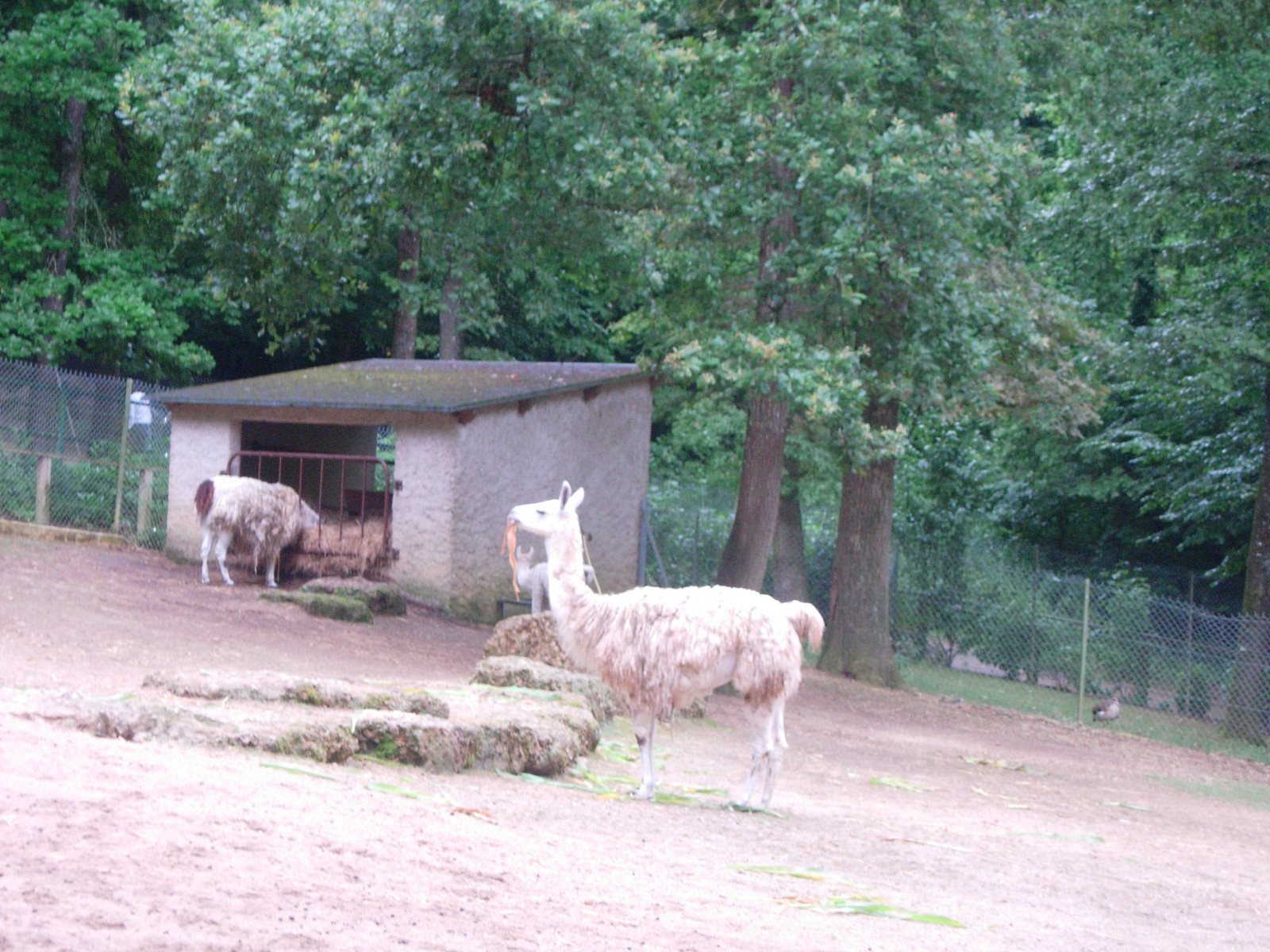In this landscape-oriented color photograph capturing a llama farm, the central focus is on two white llamas amidst a rustic setting. The foreground features one llama standing with its face turned to the left, displaying its long, shaggy white hair and a long orange item hanging from its mouth. This llama stands on a patch of brown dirt, surrounded by scattered bales of hay.

To the left, a small stone lean-to with a black roof houses another bale of hay. The structure, adorned with some leaves, has a red barrier gate at its opening, through which the second llama is feeding. This llama's head is stuck through the gate bars to access the hay inside. The farm is enclosed by a silver chain link fence, and in the distance, several large, green-leaved trees provide a lush backdrop.

Additionally, among the grass and leaves, a duck can be seen peering in from the right corner of the image. The scene combines elements of photographic realism with a representational view of a tranquil farm environment.